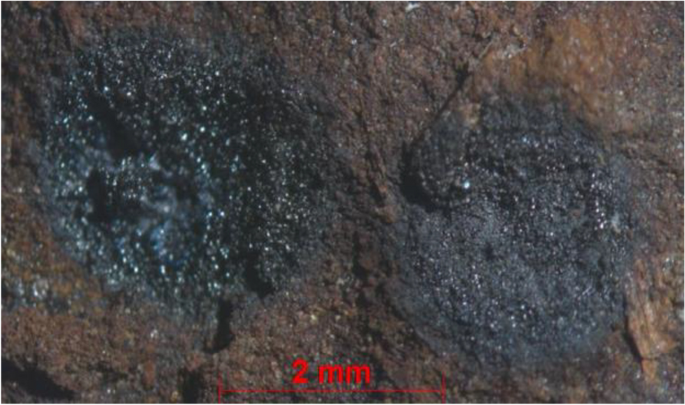This landscape-oriented color photograph shows a dark brown iron or rock surface, featuring two distinct black marks side by side. The mark on the left side is grainy and diffused with a grayish liquid-like middle, while the mark on the right side is more defined and dry. Both black marks have somewhat circular and spiral patterns, with some spirals resembling numbers, such as three and eight. Serving as a detailed backdrop, the iron or rock surface extends across the entire image, creating a textured contrast that highlights the black marks.  At the bottom of the image is a red horizontal line indicating a scale of 2 millimeters, flanked by vertical lines on each end for precise measurement.